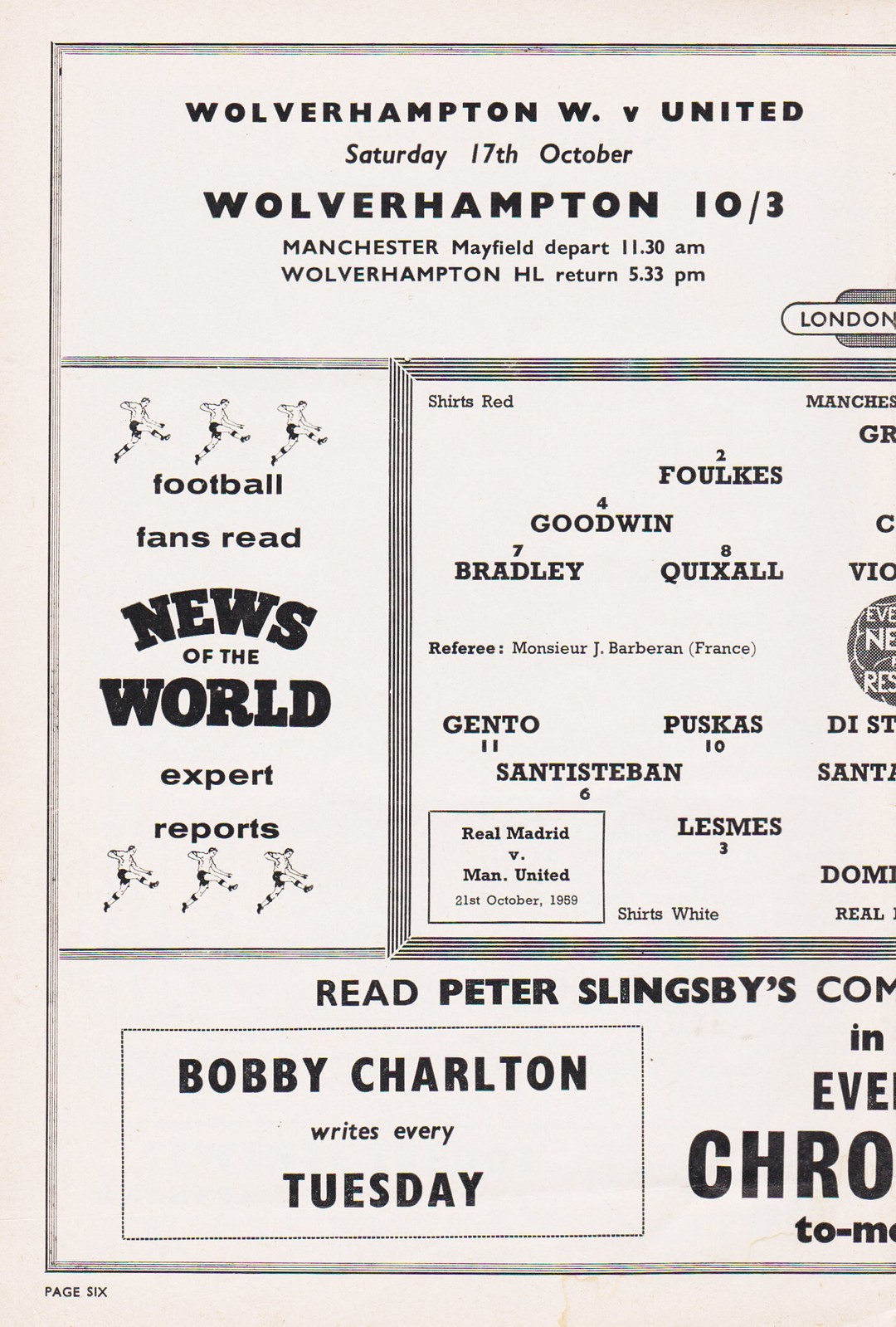The image appears to be a scanned portion of a British soccer program, specifically from a page in a pamphlet or magazine. The visible section, likely the left half of a double-wide sheet, features a central title declaring "Wolverhampton W Vs United" for a match scheduled on "Saturday, October 17th." Below the title are details about travel arrangements, specifically "Wolverhampton 10-3," suggesting an event time, and "Manchester Mayfield depart 10:30 a.m., Wolverhampton return 5:33 p.m."

On the left side of the sheet, there's an advertisement encouraging "football fans to read News of The World expert reports." The sheet is pinkish with black text, showing a central arrangement of player names: Goodwin, Quicksault, Bradley, Gento, Puskis, Santa Esteban, and Lesmes, possibly indicating their positions on the field. Below this, another box states "Real Madrid versus Manchester United."

An advertisement along the bottom reads "Read Peter Slingsby’s comments" (truncated) and mentions "Bobby Charlton writes every Tuesday," alongside a probable reference to the "Evening Chronicle." The very lower left corner features a barely legible page number, hinting this is from the center of the publication.